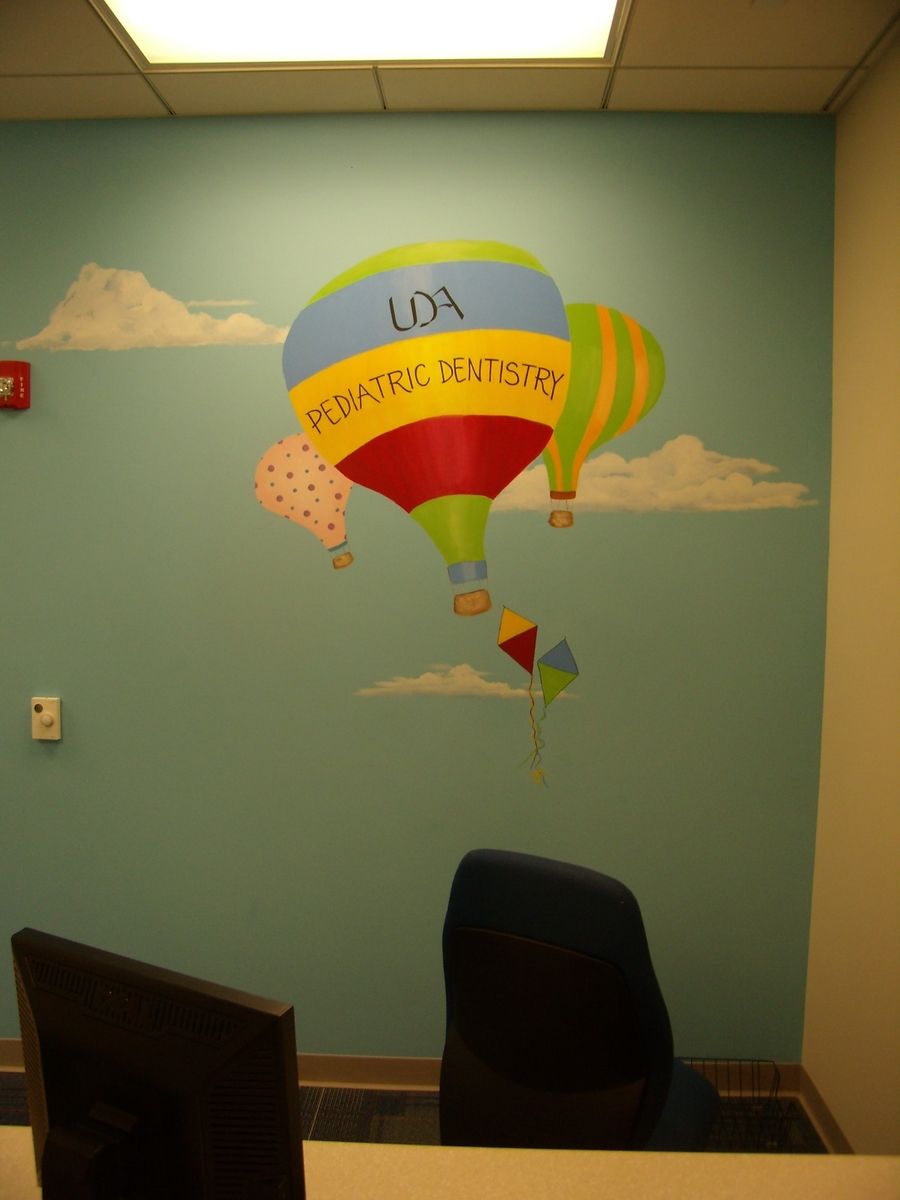The photograph is of an accent wall inside a pediatric dentist's office, featuring a hand-painted mural. The wall is bright sky blue, adorned with three fluffy clouds and three hot air balloons floating amidst the sky, accompanied by two colorful kites. The smallest hot air balloon, located to the left, is light pink with red polka dots. The large central hot air balloon boasts stripes in green, light blue, yellow, red, and green, with the text "UDA Pediatric Dentistry" prominently displayed. To its right, a medium-sized hot air balloon features vertical stripes of green and yellowy orange. The foreground includes part of a beige-colored desk and a black computer monitor on the left side. A black computer chair is also visible. Additional elements in the room include a dial for adjusting the AC, a fire alarm partially cut off on the left, ceiling tiles, a square office light, and two small chairs for children against the adjacent solid white wall.